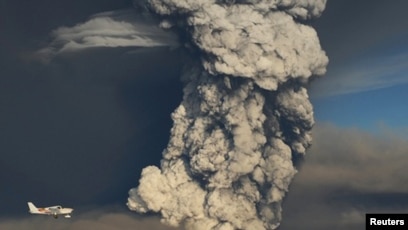The image captures a dramatic scene featuring a small white airplane, identifiable by a possible red marking on its tail fin, flying perilously close to a massive smoke cloud, likely from a volcano erupting. The airplane is positioned in the bottom left-hand corner, heading towards the enormous gray and black plume that dominates the scene. The left half of the image is enveloped in dark, almost black sky, adding to the foreboding atmosphere. To the right of the shadowy cloud, there's a narrow strip of blue sky, flanked by a mix of brownish and blackish-gray hues. Hazy clouds further populate the upper-right and bottom-right corners of the image. The photograph, credited to Reuters (R-E-U-T-E-R-S), carries a sense of urgency and danger, highlighting the stark contrast between the tranquil sky and the menacing smoke plume rising from the ground.